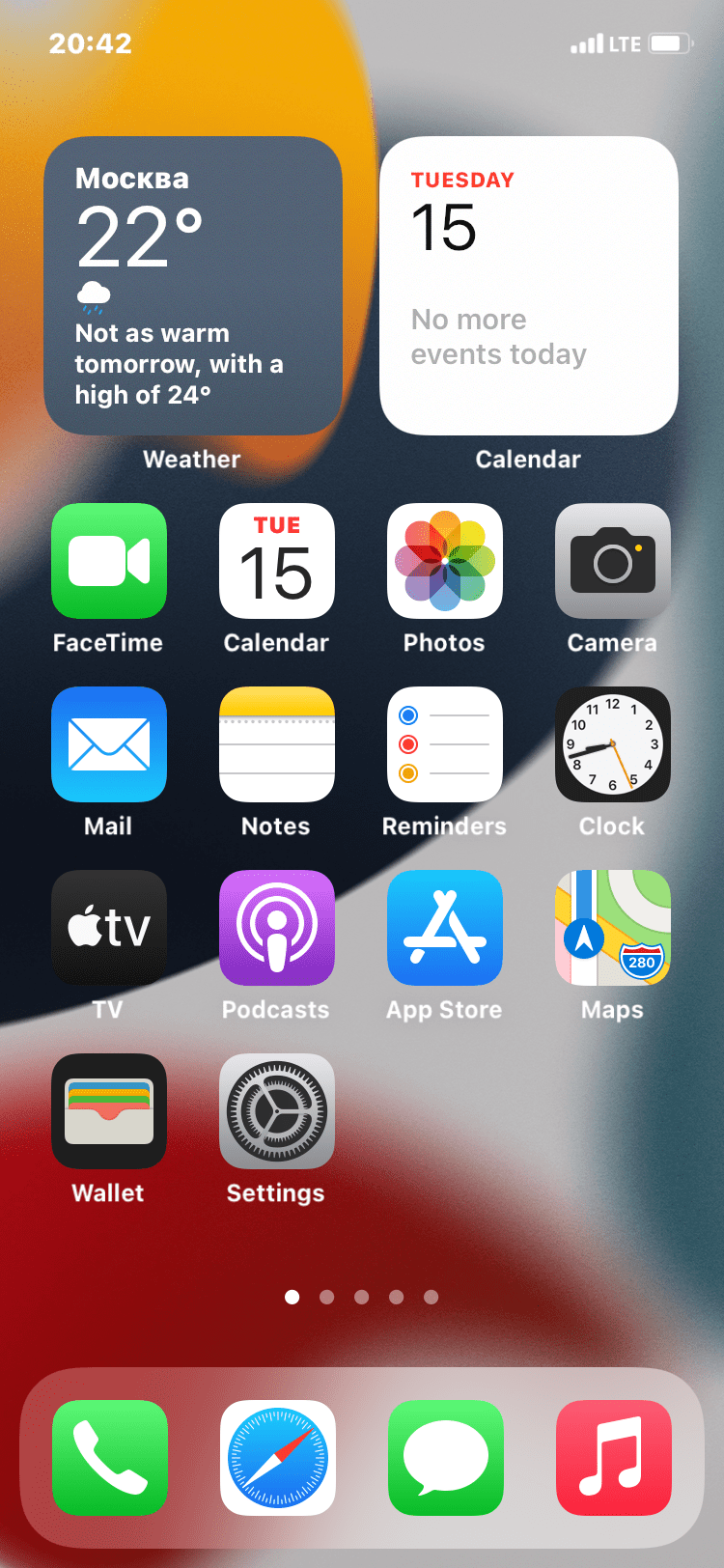The screenshot captures the home screen of a smartphone, displaying an array of vividly swirling colors as the background. In the lower right and left corners, shades of red can be seen, while the upper left is enveloped in a warm orange. The central portion features a striking black and white blend, transitioning to a bluish-green hue on the right side, creating a dynamic and eye-catching visual.

In the upper left corner of the screen, the time is displayed as 20:42. The upper right corner shows standard icons for LTE signal strength and battery life, providing essential information at a glance. Below these, there is an Eastern European text indicating the weather conditions, which shows a cloud symbol with rain and a temperature of 22 degrees. A note beneath these icons states, "Not as warm tomorrow, with a high of 24 degrees Celsius," indicating the upcoming weather forecast.

Further down, the date is marked as "Tuesday the 15th," with a notification that reads, "No more events today," underlining the user's calendar status. 

The home screen features a grid of app icons, including FaceTime, Calendar, Photos, Camera, Mail, Notes, Reminders, Clock, TV, Podcasts, App Store, Maps, Wallet, and Settings. At the very bottom, prominently highlighted, are the primary app shortcuts for Phone, Compass, Messages, and Music.